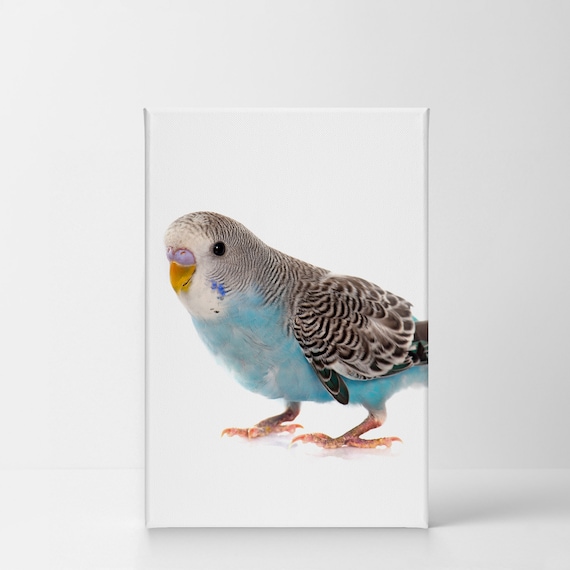The image depicts a parakeet standing against a solid white background, possibly a white vertical rectangle like a canvas or tablecloth. The parakeet’s head and back display a mix of gray and black feathers, with the wings being slightly darker, incorporating more black than white. Its beak is yellow with a hint of purple at the base, surrounded by white feathers extending to the neck area. The bird's underbody is adorned with striking turquoise blue feathers. The parakeet has orange webbed feet, dark black eyes, and casts a shadow to the right. This detailed portrayal highlights the contrast of the vibrant bird against the stark white backdrop.